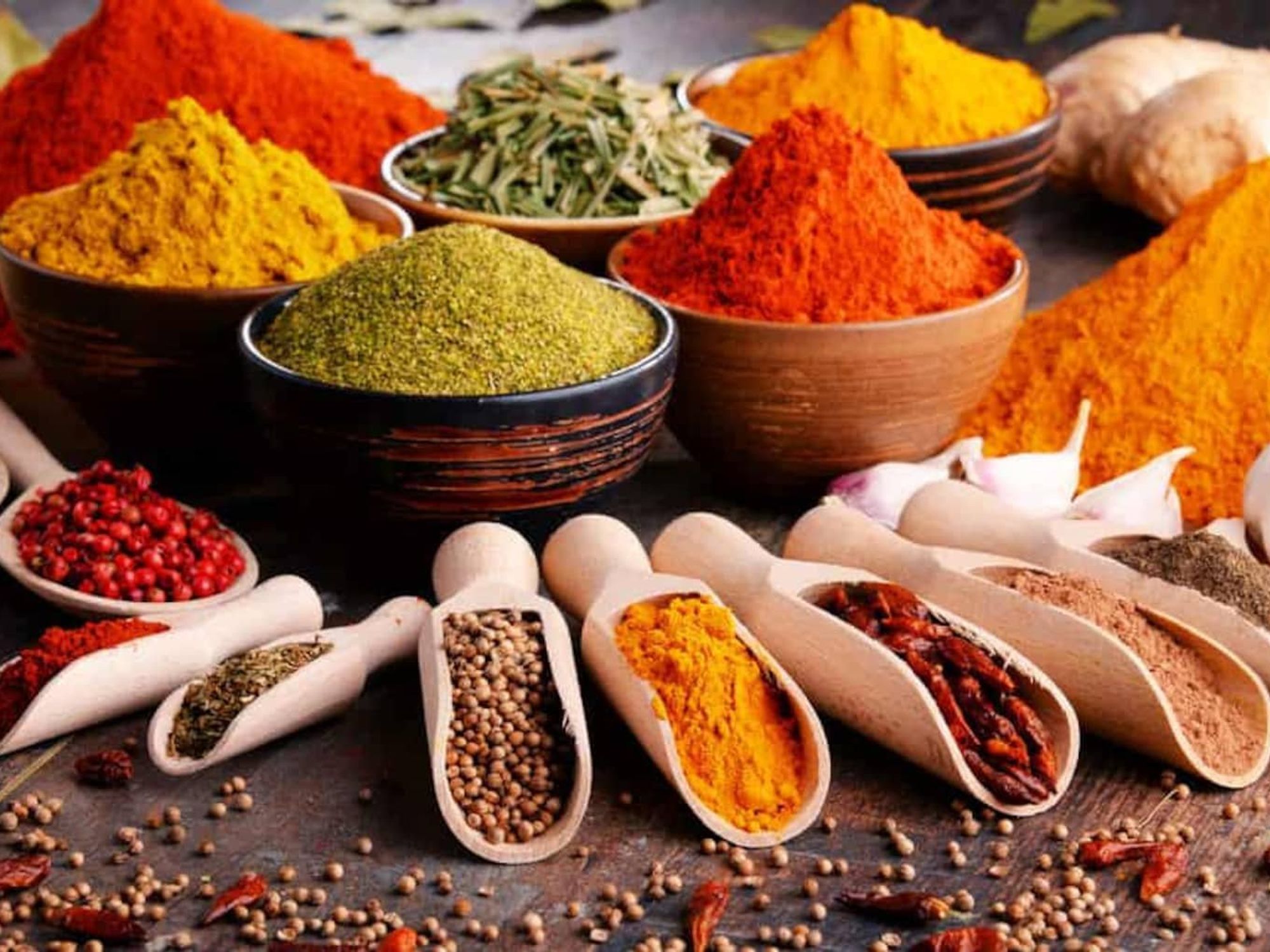This close-up, well-lit photograph showcases a vibrant and detailed array of spices, meticulously displayed with scoops and bowls on a dark brown wooden table. On the far back left, there's a large pile of orangish-red spice, resembling a small hill. Adjacent to that, to the right, sits a ceramic bowl partially in view, dark brown, filled with a light green garnish or herb. Next in line, a metal bowl adorned with black and silver stripes contains a bright orange spice. To the right of this are two unidentifiable objects, possibly a light brown-red color. 

In the forefront of the orangish-red pile, a yellow spice sits atop another ceramic bowl, with only its white interior visible. Directly in front of this bowl, there are two more spice bowls: one black with brown stripes, filled with a granule light green spice, and the other light brown with darker stripes, holding a high pile of red spice. Beside these, on the left, a scoop holds small, deep red berries.

Arranged sequentially from left to right, there are several scoops—some funneled—filled with various spices: red spice, green spice, small circular light brown pieces, orange spice, dried red chilies with maroon accents, brown spice, and lastly, a mix of gray and black spice. These scoops are interspersed with scattered small circular light brown pieces and dried chilies, adding to the rich and colorful tapestry of spices.